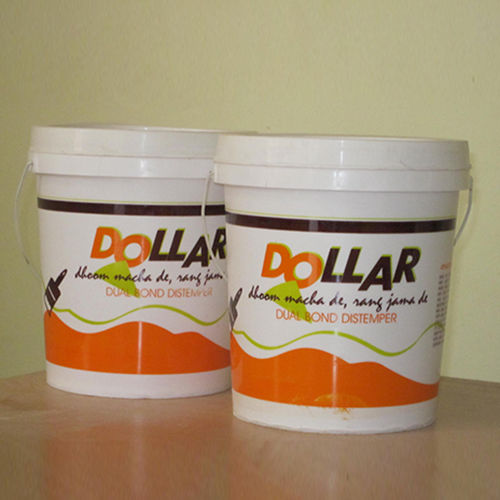The image features two white plastic buckets placed side by side on a table against a white wall. Both buckets bear the same label displaying a prominent word "DOLLAR," with the first two letters in orange and the last four in black, set against a black stripe near the top. Below this branding, there is text in a different language, identified as Spanish, followed by the phrase "dual bond distemper." Beneath this text is a squiggly green line, and at the very bottom, there are orange shapes resembling hills with a paintbrush positioned above them. The buckets appear to be related to construction or painting, as suggested by the presence of the paintbrush and the term "distemper," which is typically used in the context of wall paint and finishes. The objects are oriented to face the camera directly, allowing a clear view of their front labels, which might indicate a professional setting, possibly a business environment.